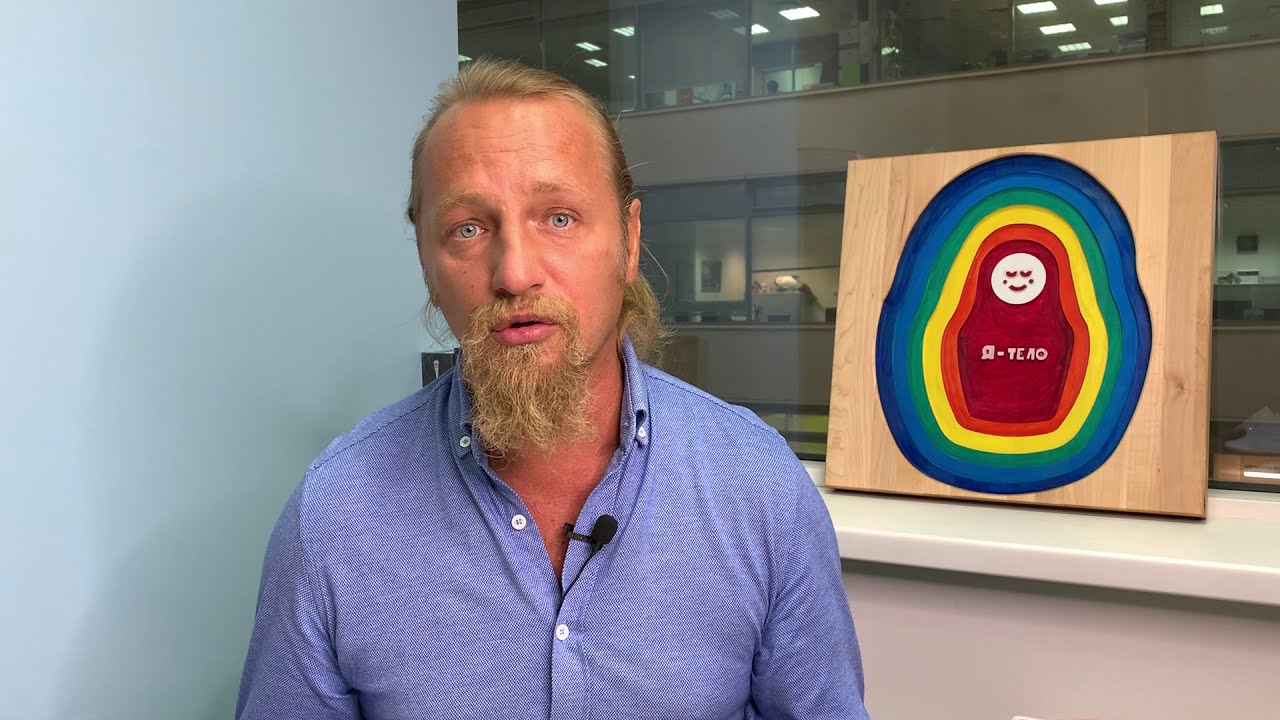In this detailed photograph, a man in a blue, casual button-up shirt with the top three buttons open is looking directly into the camera. A small black lapel microphone is pinned to his shirt, suggesting he is possibly engaged in an announcement or interview. The man appears to be around 35-40 years old, with light-colored eyes and a receding hairline, though his longer blonde hair is tied back into a ponytail. His facial hair consists of a scruffy goatee and a mustache. To his right, placed on a windowsill, there is a wooden board featuring a colorful depiction of a matryoshka doll, characterized by a small red doll with a white, smiling circular face at the center, and surrounded by concentric color rings of orange, yellow, green, turquoise, and blue. This wooden artwork rests against a glass window, behind which dimly lit office spaces with indistinct figures can be seen. The scene captures a blend of personal detail and a hint of activity in the background.